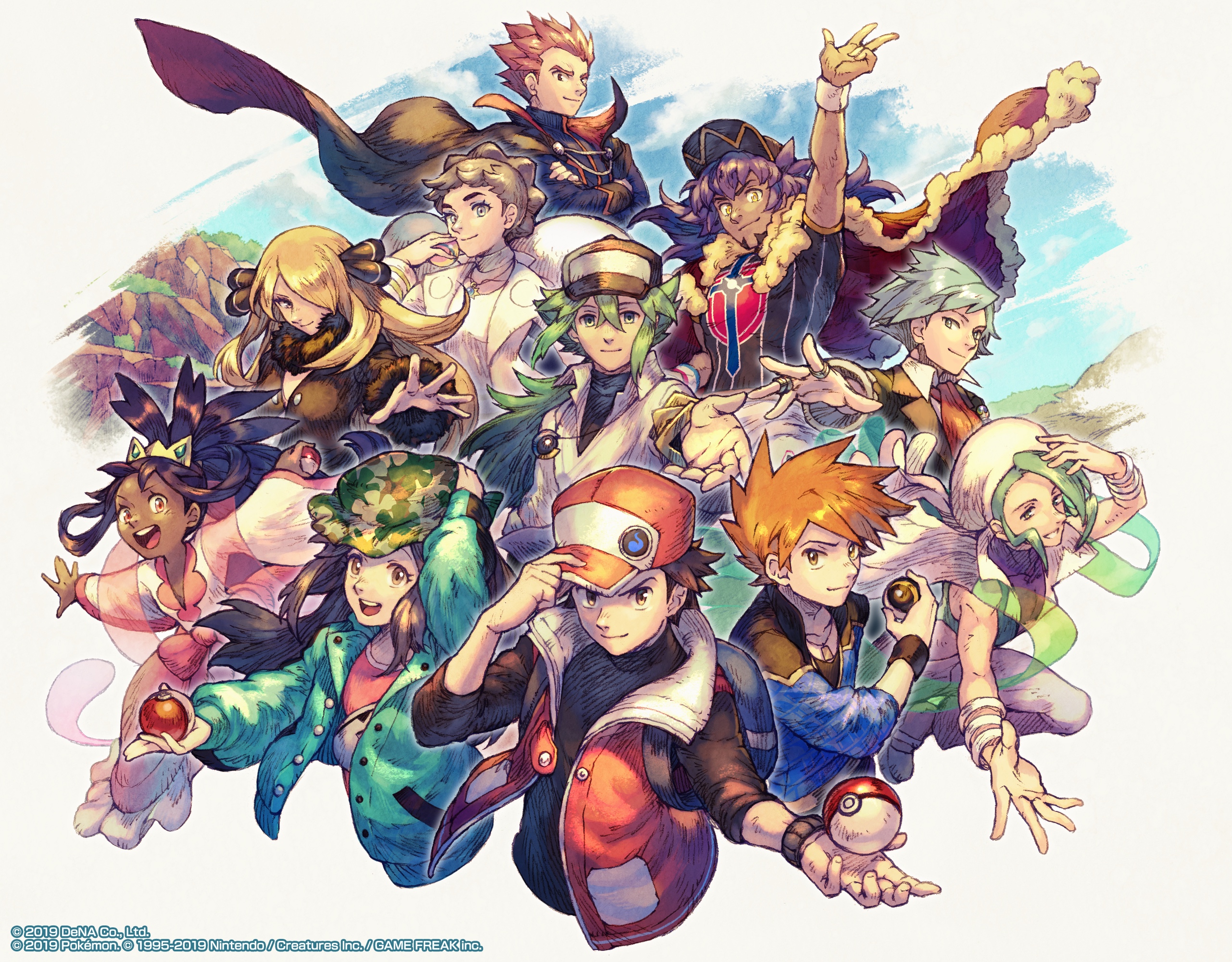This detailed illustration, possibly created with watercolor or inked and colored with markers, depicts a scene that closely resembles anime, featuring characters from the popular Pokemon series. At the center of the image is Ash Ketchum, identifiable by his red and white hat and matching vest, holding a Pokeball in one hand while the other touches his hat. Flanking him are various other recognizable Pokemon characters: to his right stands a girl with bluish-green hair and a Pokeball, and to his left, a girl with brown hair also holding a Pokeball. The background showcases a blue sky with some rocky hills on the left and mountains on the right, with a white border framing the image. Behind Ash and the two girls, about ten other anime characters fan out, each extending a hand forward as if poised to throw a ball. At the lower left of the image, the text reads "2019, Dina Co Ltd, 2019 Pokemon, 1995, 2019 Nintendo Creatures Inc. Game Freak." The detailed and vibrant artwork not only captures the essence of the Pokemon series but also suggests a blend of various anime styles, adding depth and vibrancy to the scene.